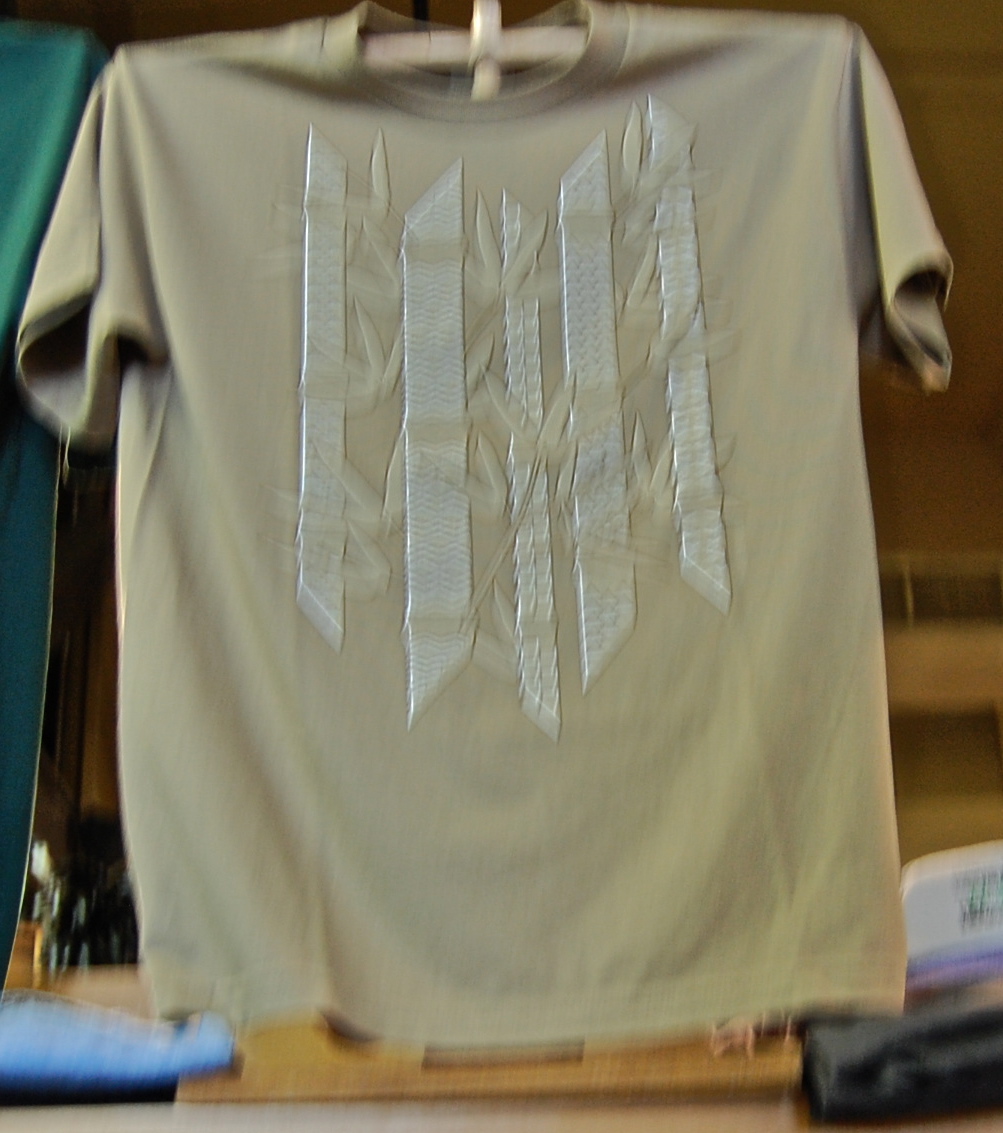This image showcases a high-quality, intricately embroidered t-shirt. The embroidery features a detailed and vibrant design, indicating meticulous craftsmanship and superior fabric quality. The artistry of the embroidery adds a unique and personalized touch to the garment, highlighting both style and elegance. The t-shirt's premium detail makes it a standout piece, perfect for those who appreciate fine embroidery work.